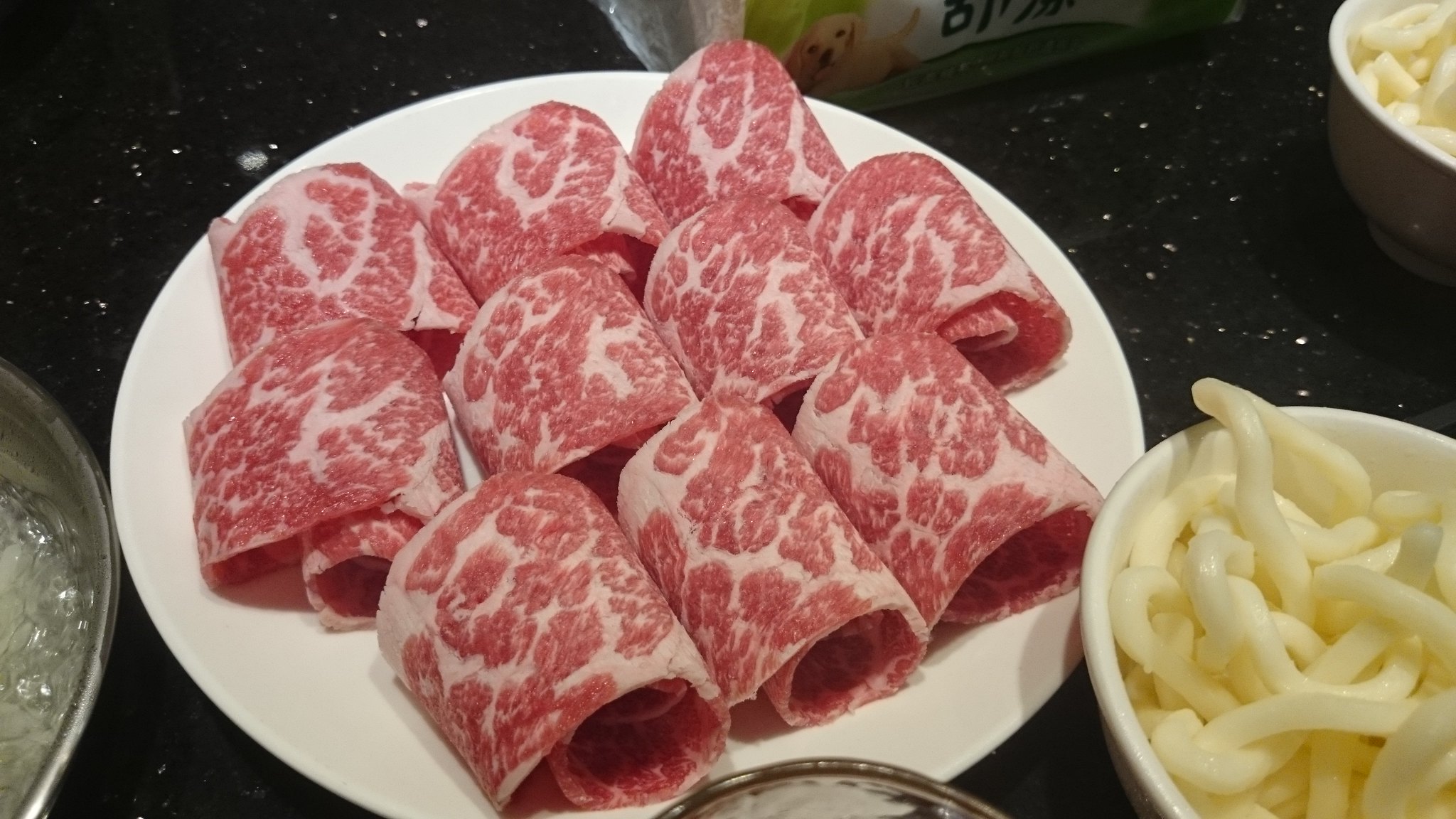The photograph captures a close-up of meticulously arranged food on a high-end black granite countertop, speckled with sparkly white flecks. Dominating the center of the image is a pristine white round plate, displaying ten neatly rolled pieces of red, marbled salami, showcasing intricate patterns of white fat. Complementing this central dish, a small silver bowl filled with ice rests to the left, while on the right, two small white bowls, possibly containing either mozzarella cheese slices or noodles, appear artfully placed—one directly to the side and another at the top right corner. Adding an interesting element, a green and white package featuring a tan golden retriever or labrador and some unreadable text is discernible near the top center of the image. Finishing the composition, an unclear clear dish is partially visible at the bottom of the frame.